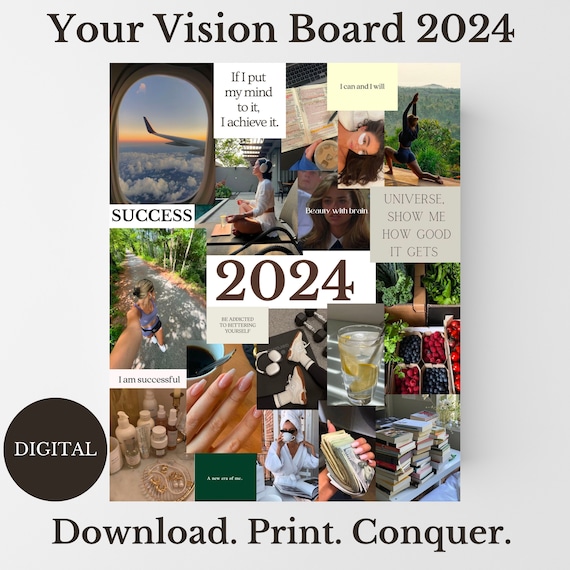This image appears to be an advertisement for "Your Vision Board 2024" on a white or grayish background. At the top, it prominently reads "Your Vision Board 2024" in black letters. Centrally, there is an example of a vision board showcasing various vibrant and inspirational images such as people outdoors, fruits, an airplane, someone practicing yoga, and a woman in a white robe. The vision board features motivational phrases including "If I put my mind to it, I achieve it," "I can and I will," "Success 2024," "Beauty with brain," and "Universe show me how good it gets," alongside images like a stack of money and books. On the bottom right of the vision board, there is a brown circle with the word “Digital” in white letters. Below the board, the text "Download. Print. Conquer." is displayed in black.